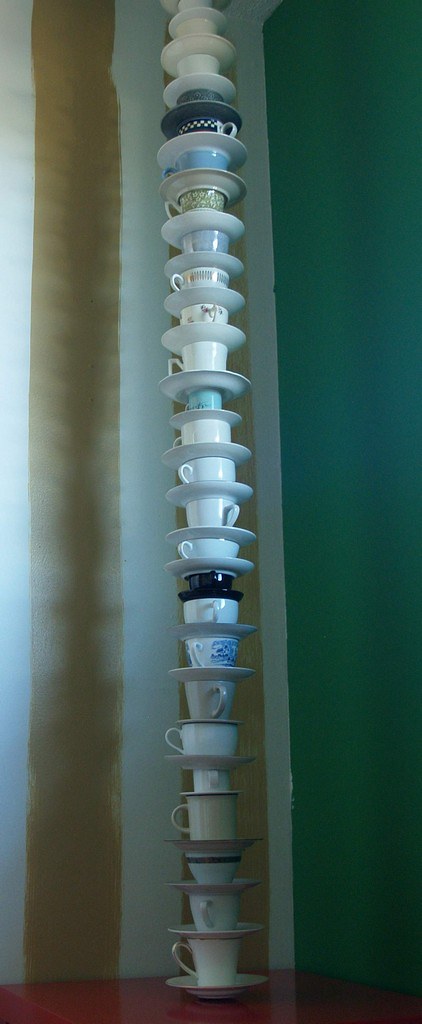In the corner of a room with contrasting walls—a striped combination of white and goldish brown on the left and a seafoam green on the right—a striking tower of teacups and saucers ascends dramatically towards the ceiling. Positioned on a corner of a wooden floor, this tower consists of about 30 to 40 delicate, porcelain china pieces, carefully alternating between saucers and teacups, creating a mesmerizing pattern of plate, cup, plate, cup. The teacups, varying in sizes and styles, predominantly feature white and beige hues, interspersed with a few floral designs, light blue, black, and even a checkered pattern. As the stack grows taller, the cups appear to increase in size. The room’s unique decor and the improbable stability of this teetering structure lend an almost surreal, Tim Burton-esque quality to the scene. This intricate and fragile tower, possibly an art installation, captures a delicate balance that defies logic, framed by soft shadows cast by an unseen light source.